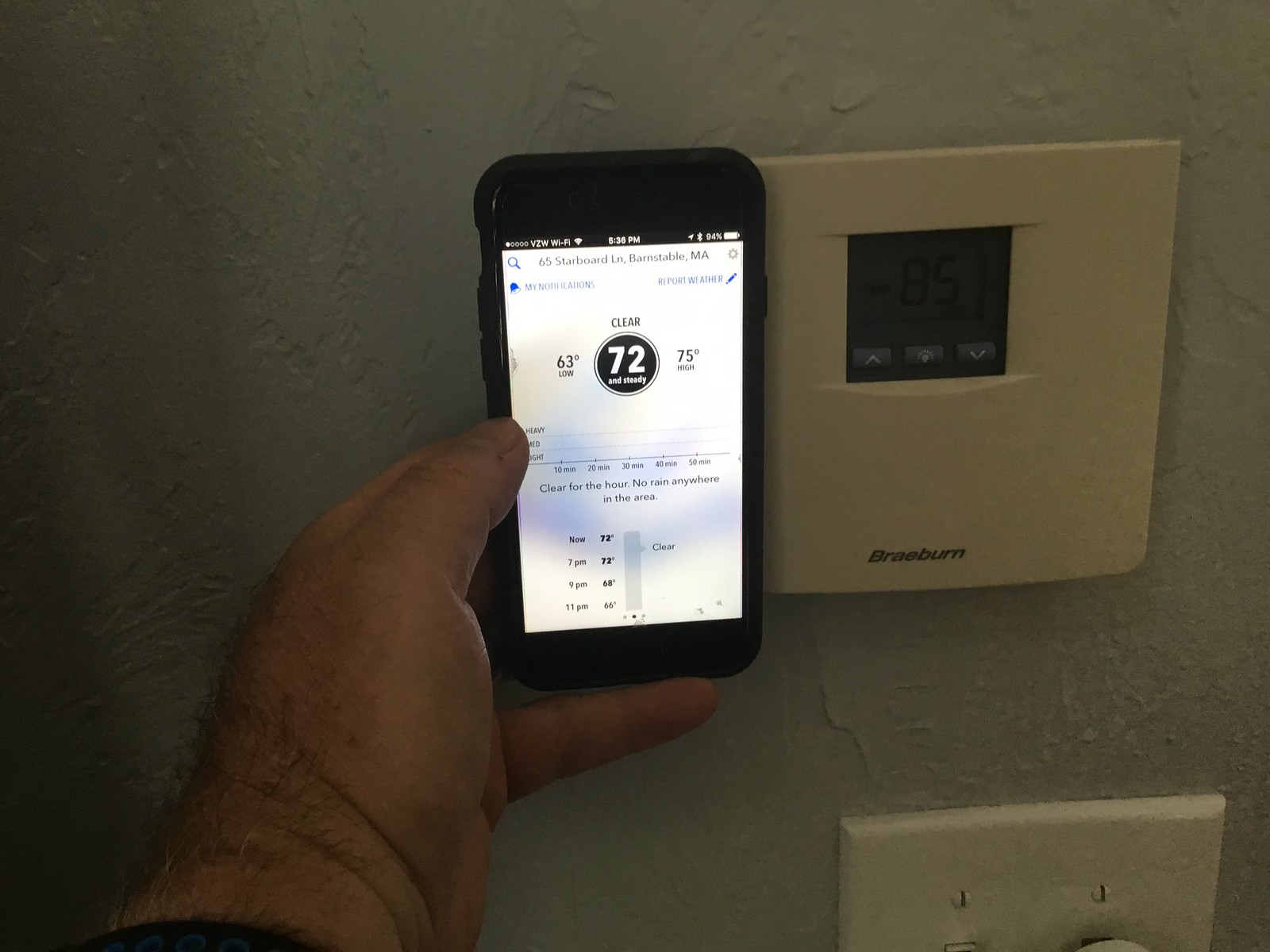In this single photograph, a light-skinned, thick, and hairy hand—suggesting it is a man's hand—holds a black smartphone. The smartphone screen, displaying a black background with a white font, shows a temperature reading of 72 degrees. The man holds the phone up to a white digital wall thermostat, which displays a contrasting temperature reading of 85 degrees. The thermostat, identified by the brand name "BRAEBU" marked on its surface, features some gray buttons and is mounted on a white wall, showing visible plaster work. Below the thermostat, there is a white light switch with a white knob. The smartphone screen also shows blurred details of the time and battery level, while a white font at the top indicates an active Wi-Fi connection.